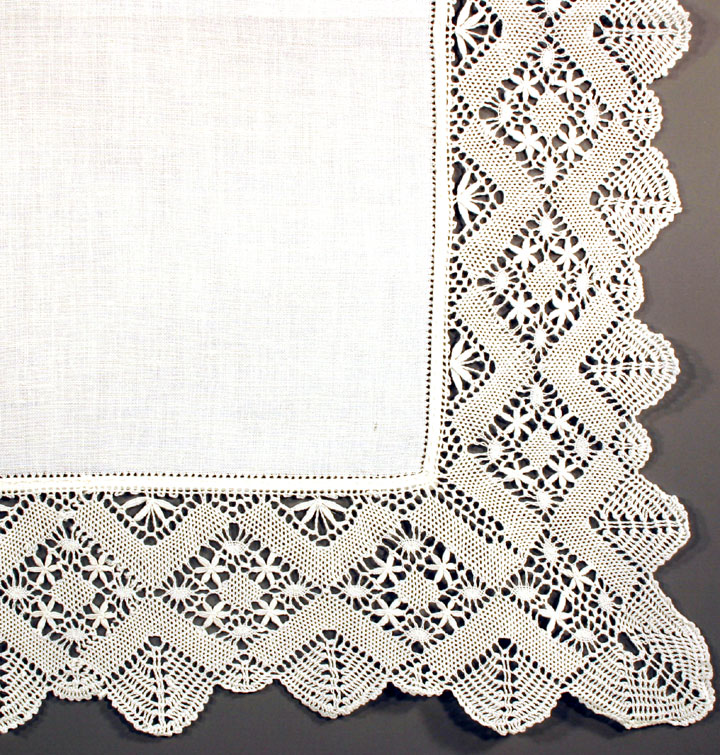The image depicts a large, magnified view of the bottom left corner of a lace placemat. The placemat features a thick, frilly lace border with a detailed pattern, incorporating see-through parts that create a delicate, airy effect with holes arranged in a pattern. The central part of the placemat is solid white, providing a sturdy area likely intended for placing tableware to protect the table underneath. The edges of the placemat are scalloped and showcase a repeating diamond pattern. The entire piece appears to be finely stitched, emphasizing both the intricate border and the solid center. The background of the image is a plain, grayish color, possibly indicating a concrete surface.